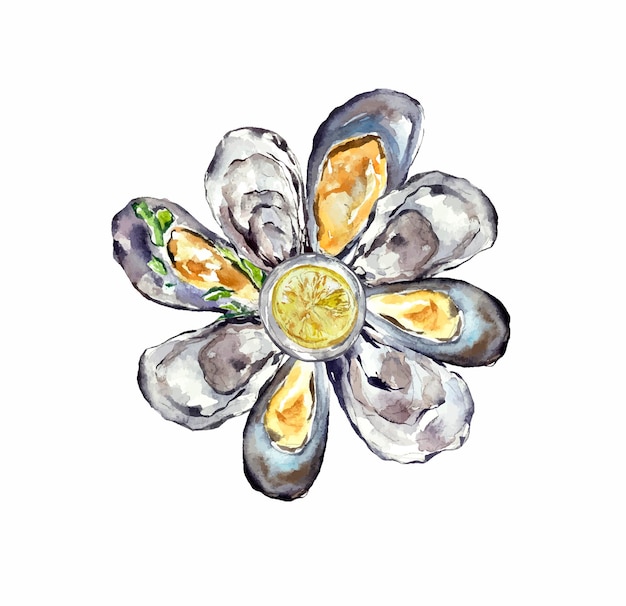This image depicts a watercolor painting from a top-down perspective, featuring eight oysters on half shells arranged in a circular, flower-like pattern. The background is completely white, bringing full focus to the oysters themselves. The shells alternate in color, with four being a silvery-gray hue and the other four a brownish tone. Positioned at approximately 10 o'clock, one oyster shell displays a hint of green, possibly resembling leaves. At the center of the circle lies a yellow, circular element that could either be a lemon or a ramekin filled with a dipping sauce, enhancing the overall composition. The painting combines intricate details and thoughtful coloration to create a striking visual reminiscent of both natural marine textures and floral symmetrical beauty.